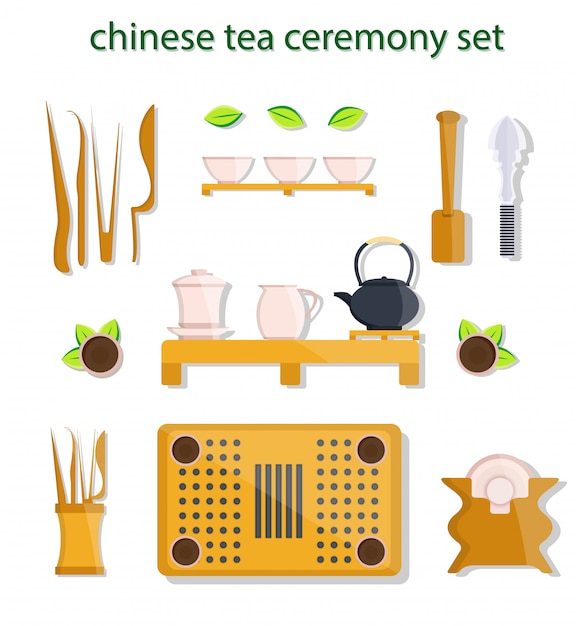A digitally drawn image displays a Chinese tea ceremony set against a white background. The top of the image features the text "Chinese Tea Ceremony Kit" in a very dark green, all in lowercase letters. The illustration is vertically rectangular without a defined border. 

The top section of the image includes three pink cups adorned with green leaves, positioned centrally. Flanking them are various bamboo-colored wooden tools, such as tongs, a fork, and chopsticks on the left, and a spatula on the right. 

In the middle section, there is a floating shelf or counter that holds two pink pitchers and a black tea kettle. 

The bottom section showcases a square mat or dish rack with numerous black holes. On this mat is a pink dish and a silverware holder containing bits of wooden utensils. The entire piece features an array of colors including light brown, black, light pink, light green, silver, and gray, contributing to a cohesive clipart or hand-drawn aesthetic.